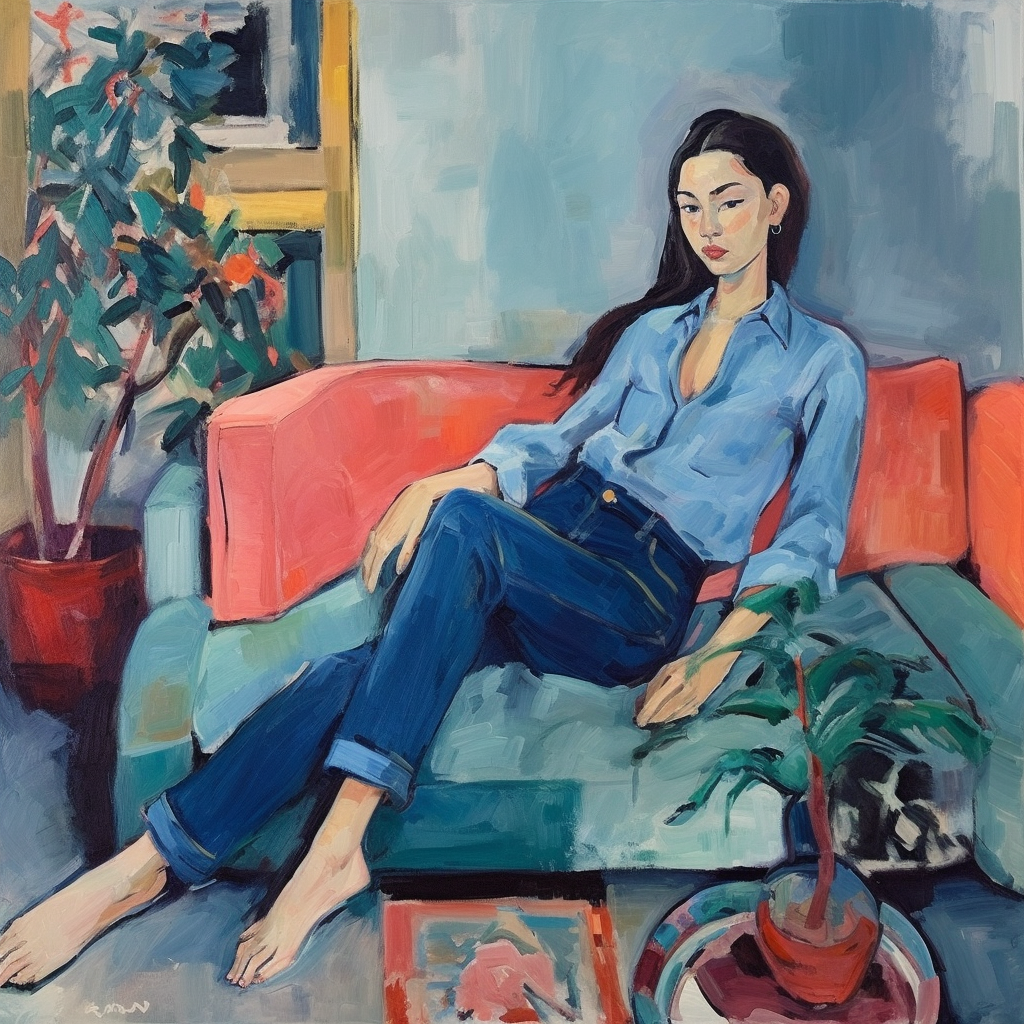The image is a detailed painting, likely done in acrylic or oil, featuring a young woman lounging diagonally on a light blue couch with blue cushions and contrasting orange pillows. She is dressed in blue jeans and a long-sleeved, button-down blue shirt with her feet firmly planted on the floor, showing that she has no shoes or socks on. The scene is set in a living room dominated by cool blue and green tones. Her long brown hair frames her relaxed posture.

To the left of the couch, a large tree or plant with green leaves and orange flowers grows out of a reddish-orange planter, positioned in front of a window with a brownish or gold frame. The background wall shares the same hue as the couch, adding to the serene atmosphere of the artwork. In the foreground, there is a small table holding a small plant and what looks like a magazine or book. A rug is visible on the floor by her feet, adding to the cozy, lived-in feel of the room. The brush strokes are visible, enhancing the texture and depth of the painting, and emphasizing the predominant bluish tones throughout.